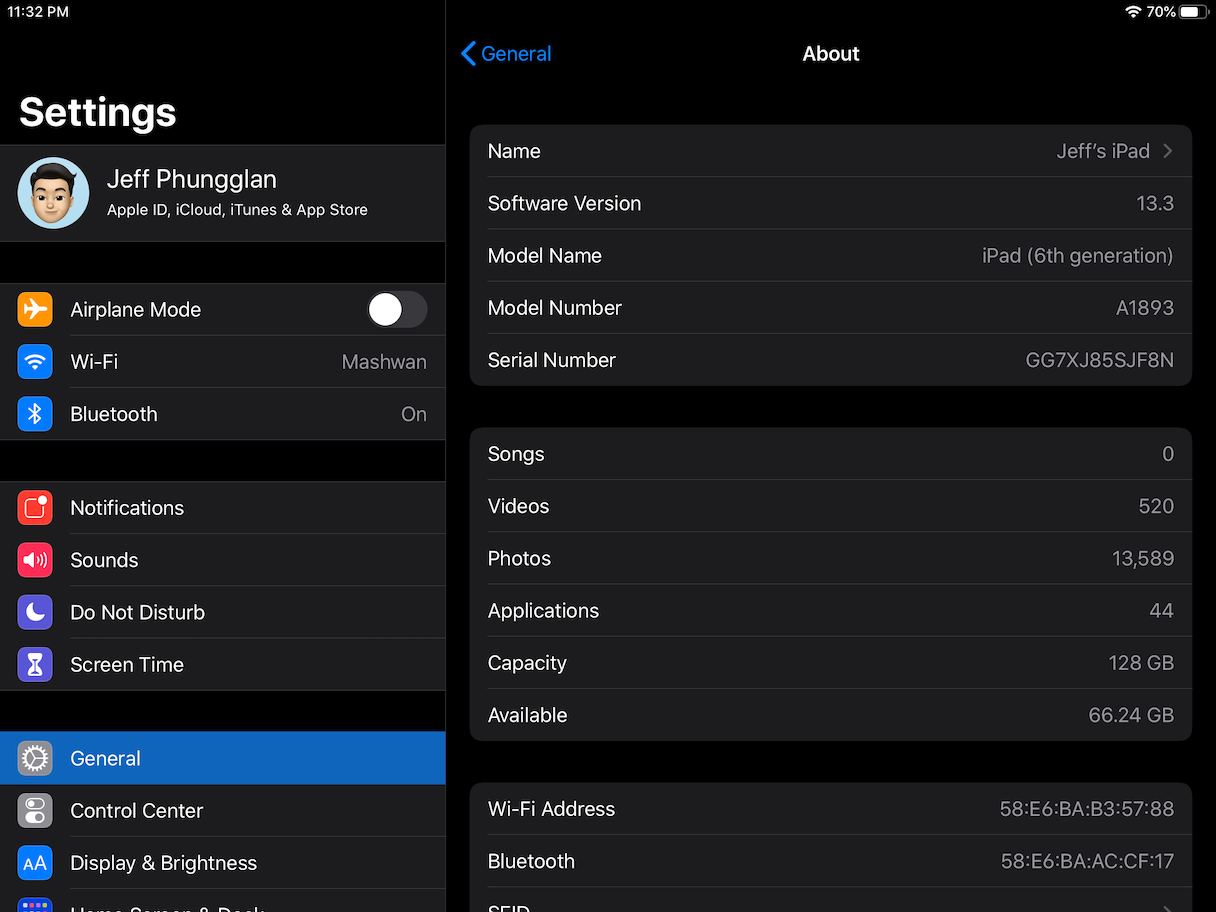This image is a detailed screenshot of a settings menu on a mobile device. The background is jet black, creating a sleek and modern look. At the top left corner of the screen, the time is displayed as 11:32 PM. In the upper right corner, there is a Wi-Fi symbol, indicating signal strength, the percentage "70%", probably showing the current battery level, and a battery icon.

On the left side of the screen, under the heading "Settings," there is a vertically aligned list of menu options. At the very top of this list is a profile picture accompanied by the name "Jeff Funglin." Below the profile picture, the text reads: "Apple ID, iCloud, iTunes, and App Store."

The menu options below are accompanied by colorful icons for easy identification. The options listed are:
- Airplane Mode
- Wi-Fi
- Bluetooth
- Notifications
- Sounds
- Do Not Disturb
- Screen Time
- General
- Control Center
- Display & Brightness

The "General" menu option is highlighted in blue, indicating that it is currently selected. This selection changes the right side of the screen to display more detailed information.

At the top center of the "General" screen, there is a heading labeled "About," with blue "General" text and a left-pointing arrow next to it, likely for navigation purposes.

Below this, there is a comprehensive list of sections extending from top to bottom, each providing specific information about the device. On the left side of this column, the sections are listed, and on the right side, their corresponding descriptions are displayed:
- Name
- Software Version
- Model Name
- Model Number
- Serial Number
- Songs
- Videos
- Photos
- Applications
- Capacity
- Available
- Wi-Fi Address
- Bluetooth

This detailed layout offers an organized and user-friendly way to navigate and manage the device's settings and information.